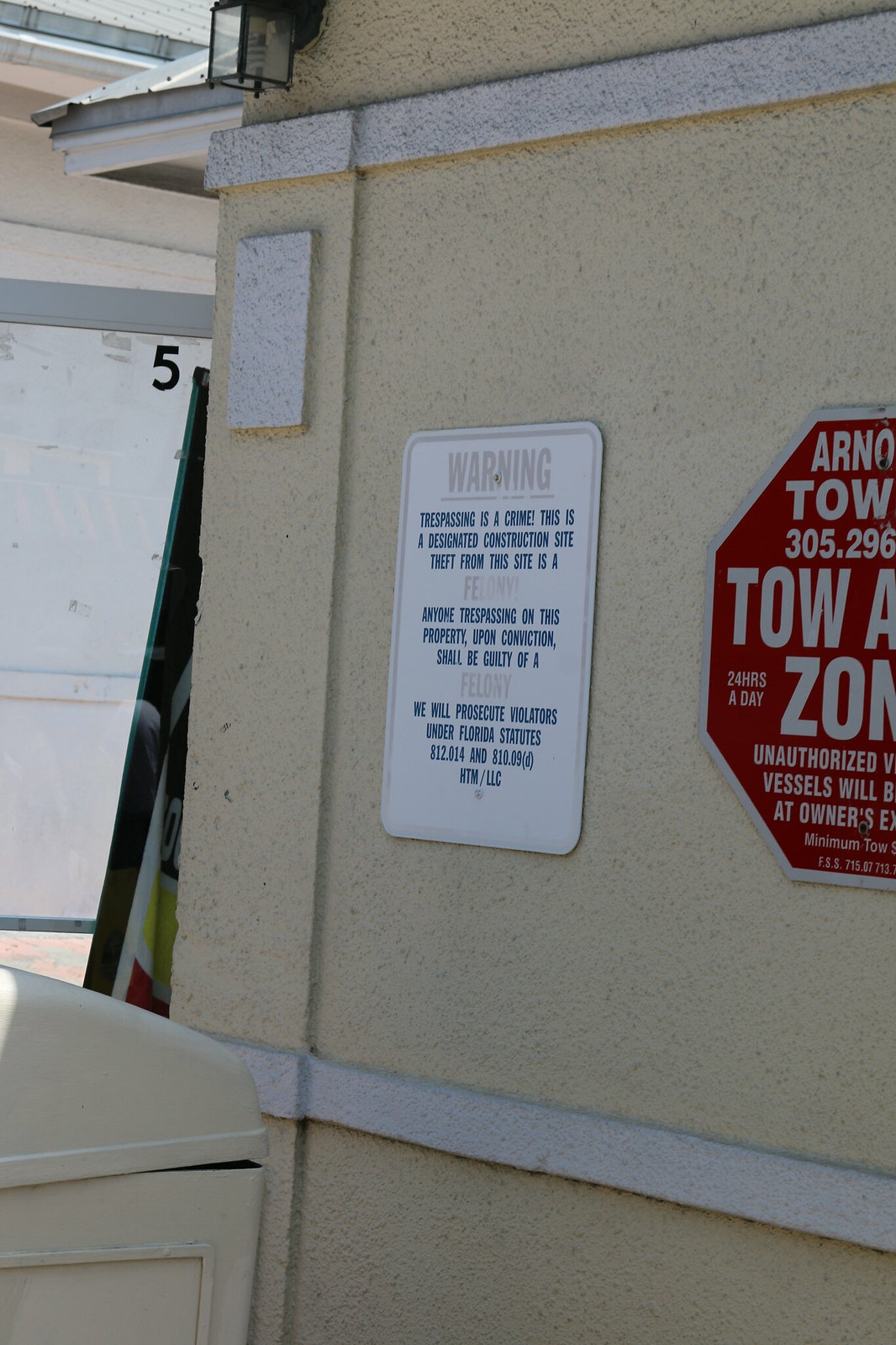This outdoor photograph captures the exterior of a beige building, possibly adjacent to a garage area. Prominently featured is a beige wall adorned with a few horizontal white boards near the top and bottom. To the lower left corner, there is a beige trash container. On the very left side of the wall, an octagonal red and white sign reads "Tow-Away Zone" and indicates that unauthorized vehicles will be towed at the owner's expense. Next to it, another sign, rectangular and white, has faded blue lettering that begins with "WARNING" and continues with "TRESPASSING IS A CRIME." It further states that this location is a designated construction site and that theft from this site is a felony. The photograph also reveals a small section of a roof at the top left corner, suggesting the building's outdoor setting. Visible in the left portion of the image, there appears to be a ladder covered by a banner and a nearby garage door marked with the number five.